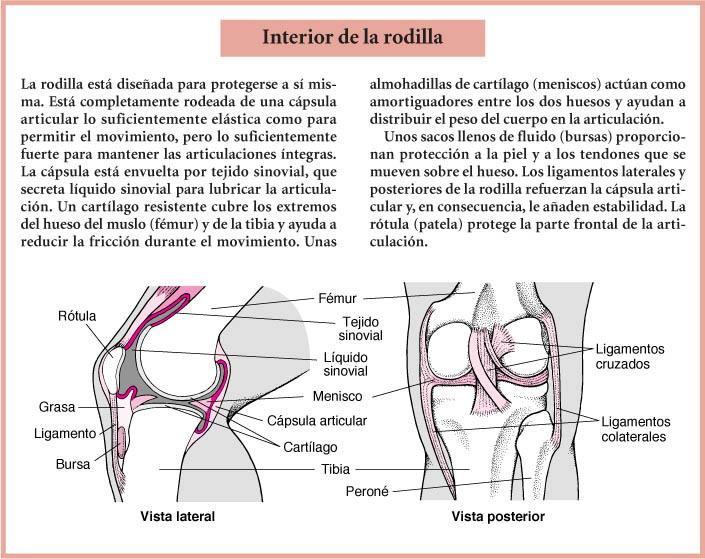The image appears to be a detailed page from a medical book or possibly a slide from a medical presentation, featuring anatomical diagrams in Spanish. It has a white background with a peach-colored border along the edges. At the top center, set against a pink rectangular background, there is a bold black header that reads "Interior de la Rodilla." Below the header, there's approximately a paragraph of Spanish text, divided into two columns.

Further down, the page features two detailed diagrams of the human knee, each labeled in Spanish. The left diagram, labeled "Vista Lateral," shows a side view of the knee with a mix of gray and white coloring for the bones and pinkish hues for the muscles. Key anatomical parts such as the femur, tibia, and ligaments are labeled with black text and connecting lines.

The right diagram, labeled "Vista Posterior," presents a posterior view of the knee, highlighting similar parts with detailed labels such as "ligamentos cruzados," "perone," and "ligamentos colaterales." The overall illustration is highly detailed, showcasing the intricate design of the knee's anatomy, with all textual labels in clear black font for easy identification.